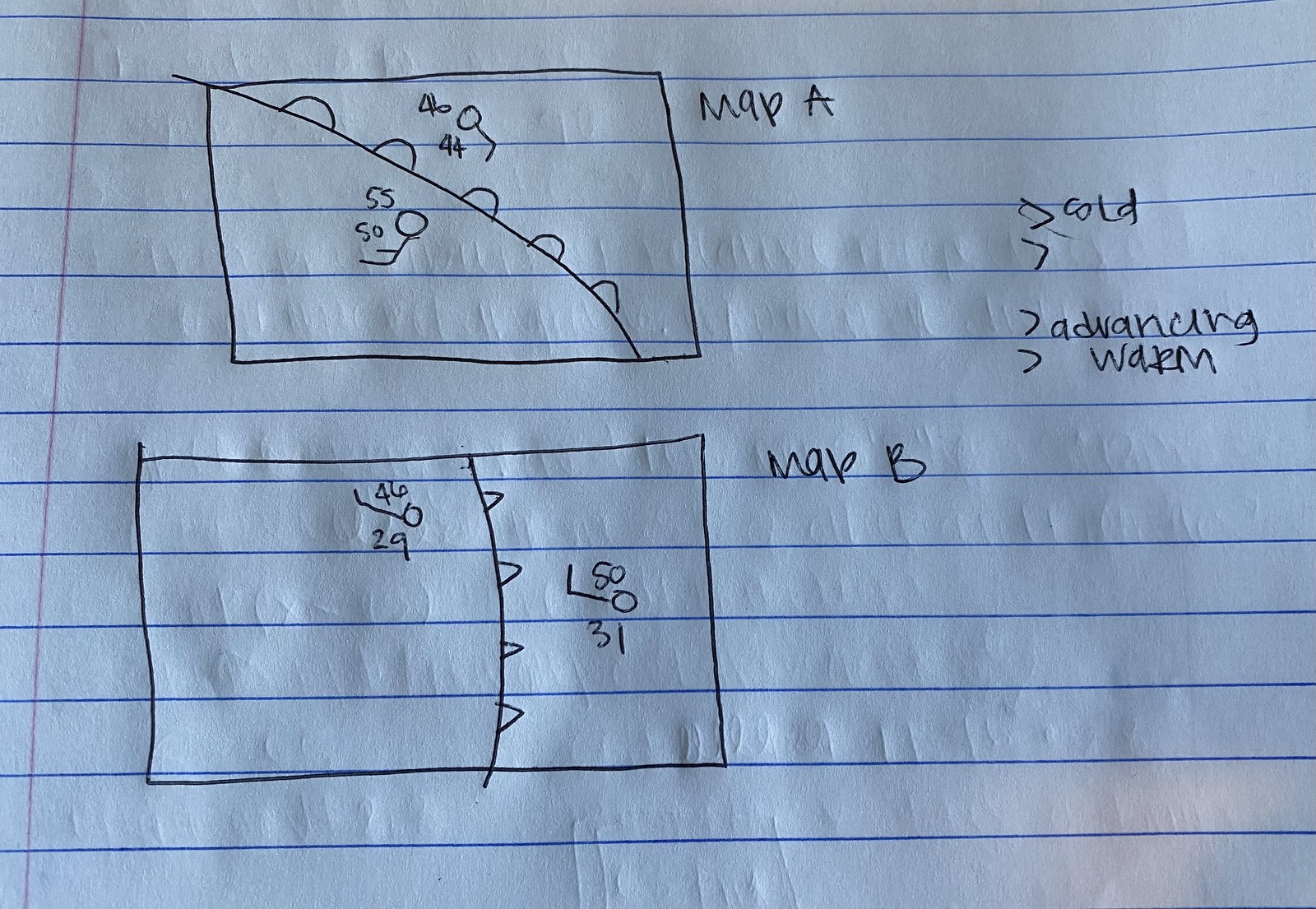In the image, two rectangular drawings are depicted on a sheet of white paper lined with thin horizontal blue lines. These rectangles, labeled "Map A" and "Map B," are aligned vertically, separated by a dividing line. 

The top rectangle, "Map A," has a diagonal line descending from the left to the right, adorned with five small, lowercase 'n'-shaped markers along its path. On the left side of this diagonal line sits a stick figure accompanied by the numbers 55 and 50. On the right side, another stick figure appears alongside the numbers 46 and 44.

The bottom rectangle, "Map B," is bisected by a vertical line featuring four rightward-pointing arrows. Situated on the left side of this line is a stick figure, separating the numbers 46 and 29. Similarly, on the right side, there is another stick figure between the numbers 50 and 31.

To the right of "Map B," the words "Cold" and "Advancing Warm" are written, offering additional context to the maps. While there is no other visible text, faint indentations from previous writings can be seen in the background on the page, hinting at earlier notations.